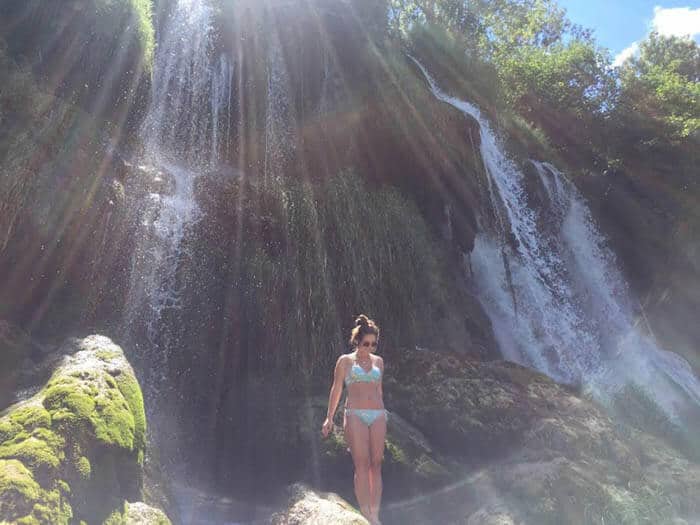The image captures a striking scene of a woman standing at the base of a colossal, roaring waterfall, with cascades of white water streaming down the mountain cliffs behind her. She has light skin and her dark brown hair is pulled up into a messy bun. She wears brown sunglasses and a detailed two-piece bikini adorned with a blend of white, light blue, green, and pink patterns. Positioned amid large rocks covered in green moss, she stands slightly out of the direct path of the rushing water, seemingly contemplating a jump as she gazes downward. The radiant sunlight illuminates the scene, highlighting the vibrancy of the setting. In the upper right corner, a bright blue sky with scattered white clouds peeks through, framed by lush green trees, adding to the natural beauty surrounding her.